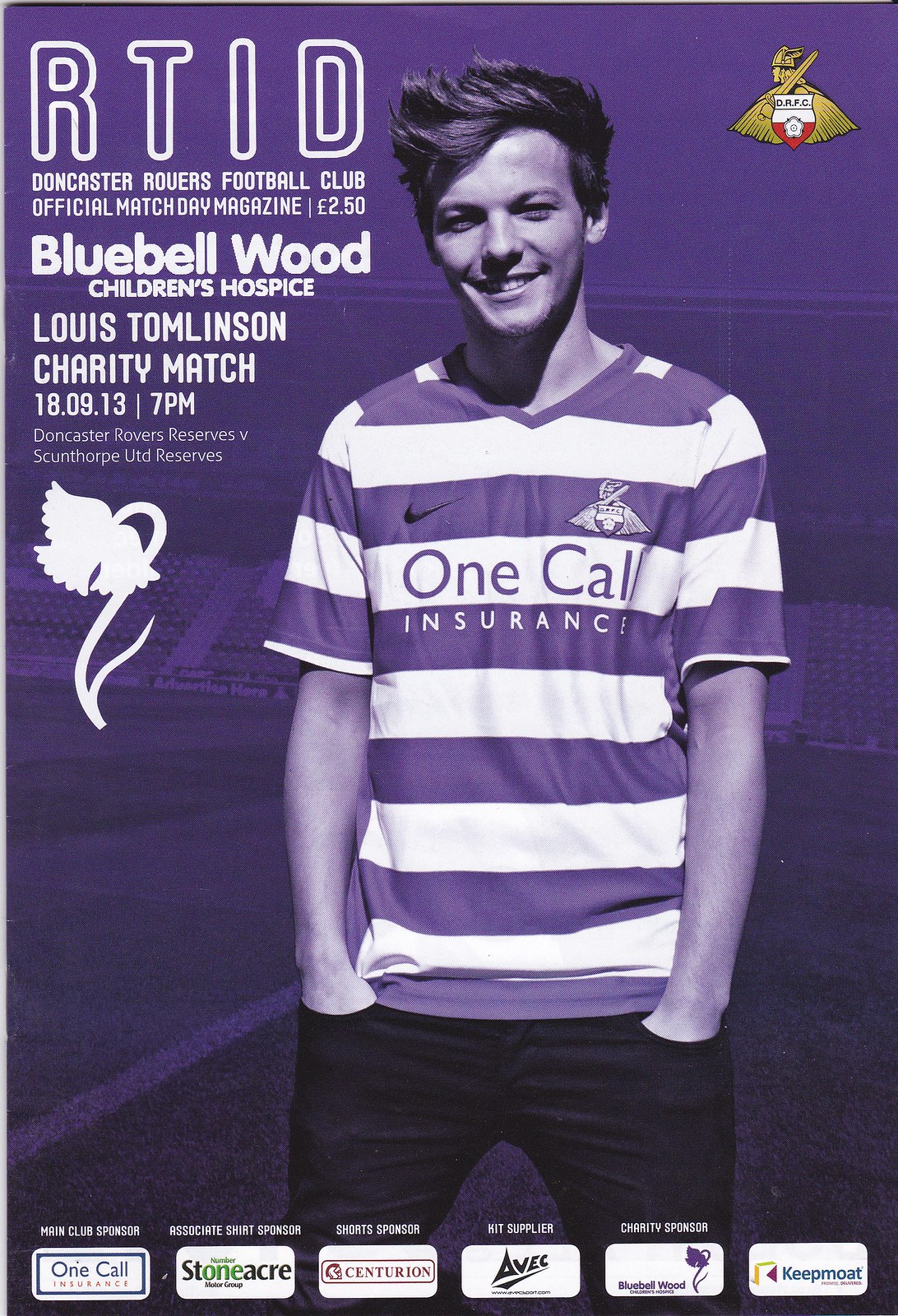The magazine cover or promotional flyer has a prominent blue tint, casting a serene blue or white hue across the entire image. Dominating the center stands a young gentleman, casually dressed in black pants with both hands in his pockets. He's wearing a v-neck, short-sleeved t-shirt adorned with blue and white stripes. On his chest, the shirt proudly displays the "One Call Insurance" logo, coupled with a checkmark and a SHIELD logo with wings on either side.

In the top left corner, several words in white font catch the eye: "RTID, Doncaster Rovers Football Club, Official Match Day Magazine, £2.50, Bluebell Wood Children's Hospice, Lewis Tomlinson, Charity Match, 18-09-13, 7 p.m." Lower down, the text confirms the charity match, specifying Doncaster Rovers Reserves versus Scunthorpe United Reserves, set for September 18th, 2013, at 7 p.m.

A subtle, white silhouette of a flower, possibly a bluebell, adds a gentle decorative touch to the image. The stadium forms a blurry backdrop, allowing the young man to stand out crisply in the foreground. The bottom section of the page features various sponsor logos, with One Call Insurance being the main club sponsor, alongside other sponsors such as Stoneacre and Centurion. The image, with its blue-wash effect, pulls together multiple elements, all contributing to promote the charity match for Bluebell Wood Children's Hospice, endorsed significantly by Lewis Tomlinson.